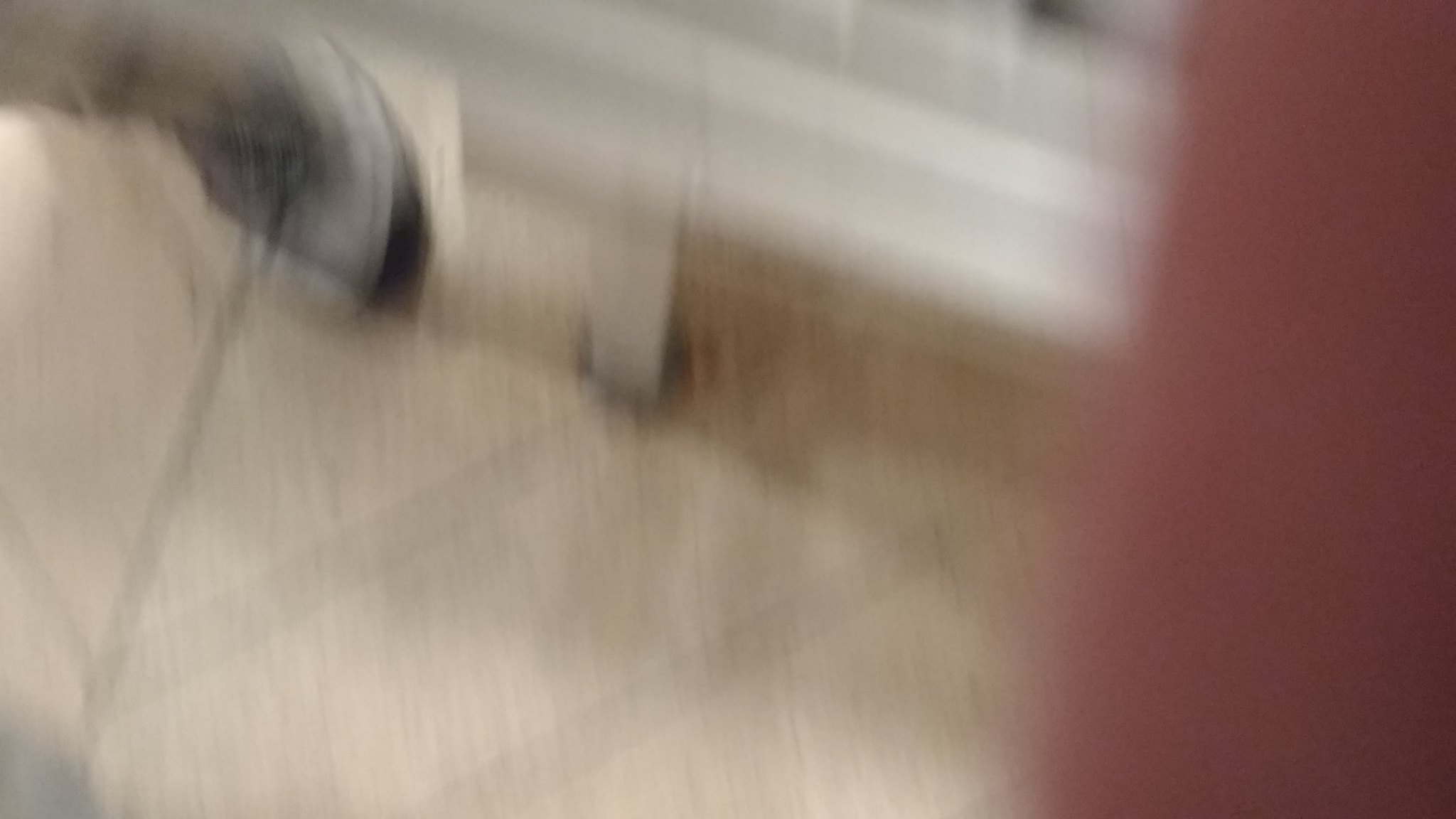This is an extremely blurry photo, primarily in a widescreen format. The majority of the image, approximately 80%, features a light tan color with faint gray lines running diagonally from the lower left to the upper right, possibly suggesting tile flooring with grout lines. On the right-hand side, there is a hint of a Caucasian skin tone—likely a finger partially obscuring the lens. Additionally, there appears to be a small wheel attached to a piece of furniture, possibly a table or cart leg, situated on what could be a tiled kitchen floor. Overall, the photo is out-of-focus, low quality, and it's challenging to determine the exact contents due to the extreme blurriness.